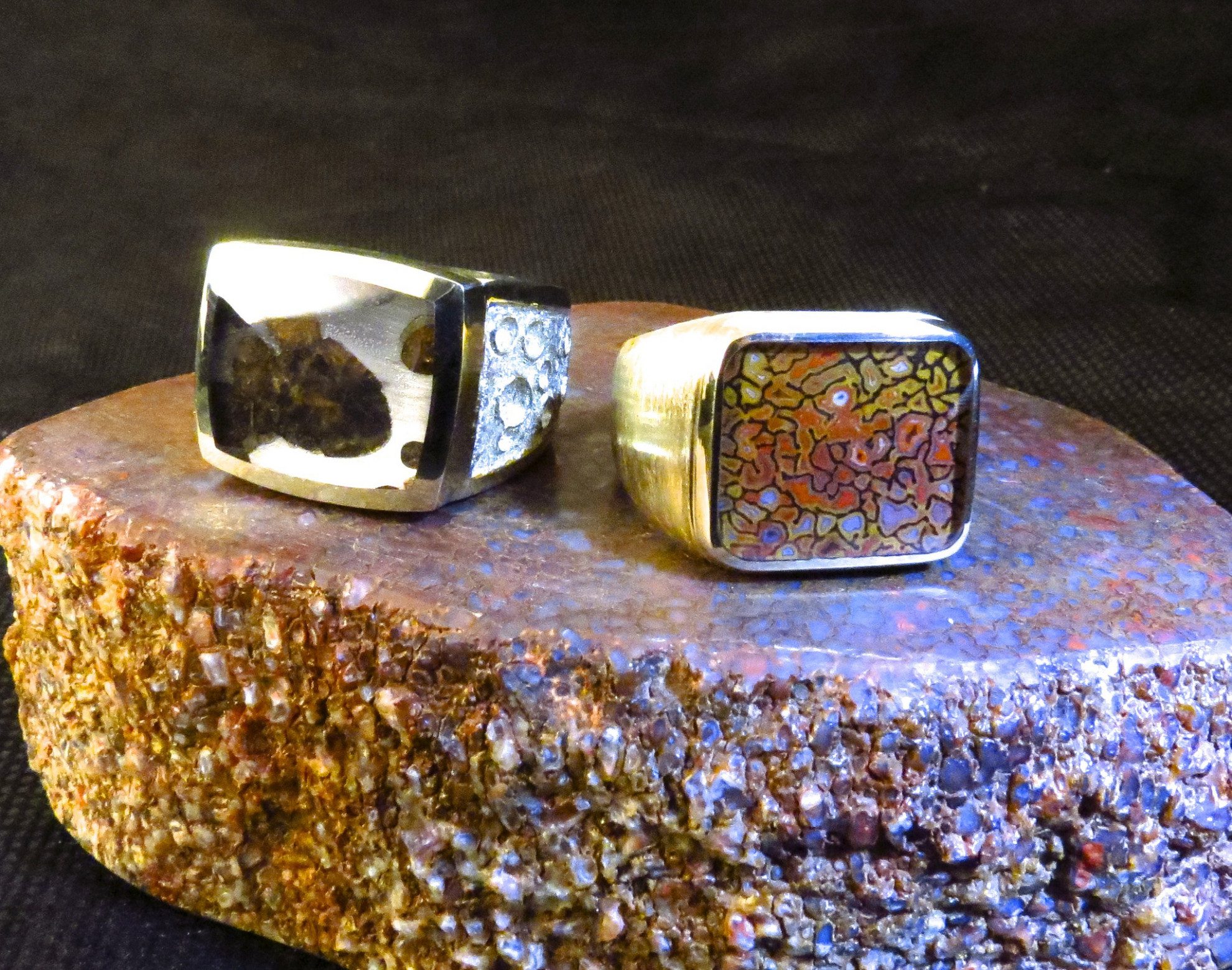The photograph features a close-up of two large rings positioned on a multi-colored stone, which in turn is placed on a black cloth background. The stone, approximately 6 inches high and 12 inches long, has a smooth top surface and a rough, unfinished edge, composed of smaller stones and pebbles amalgamated into a single, larger piece. On this smooth surface rest the thick rings, with faces reminiscent of an Apple Watch. 

The ring on the right appears to be gold, adorned with a colorful design that mirrors the pastel shades of the stone—purples, yellows, and oranges. The ring on the left contrasts with a combination design: it features a white stone element on its edge and a silver and copper pattern on its face. The overall setup accentuates the vibrant hues and intricate details of both the rings and their supporting stone platform.